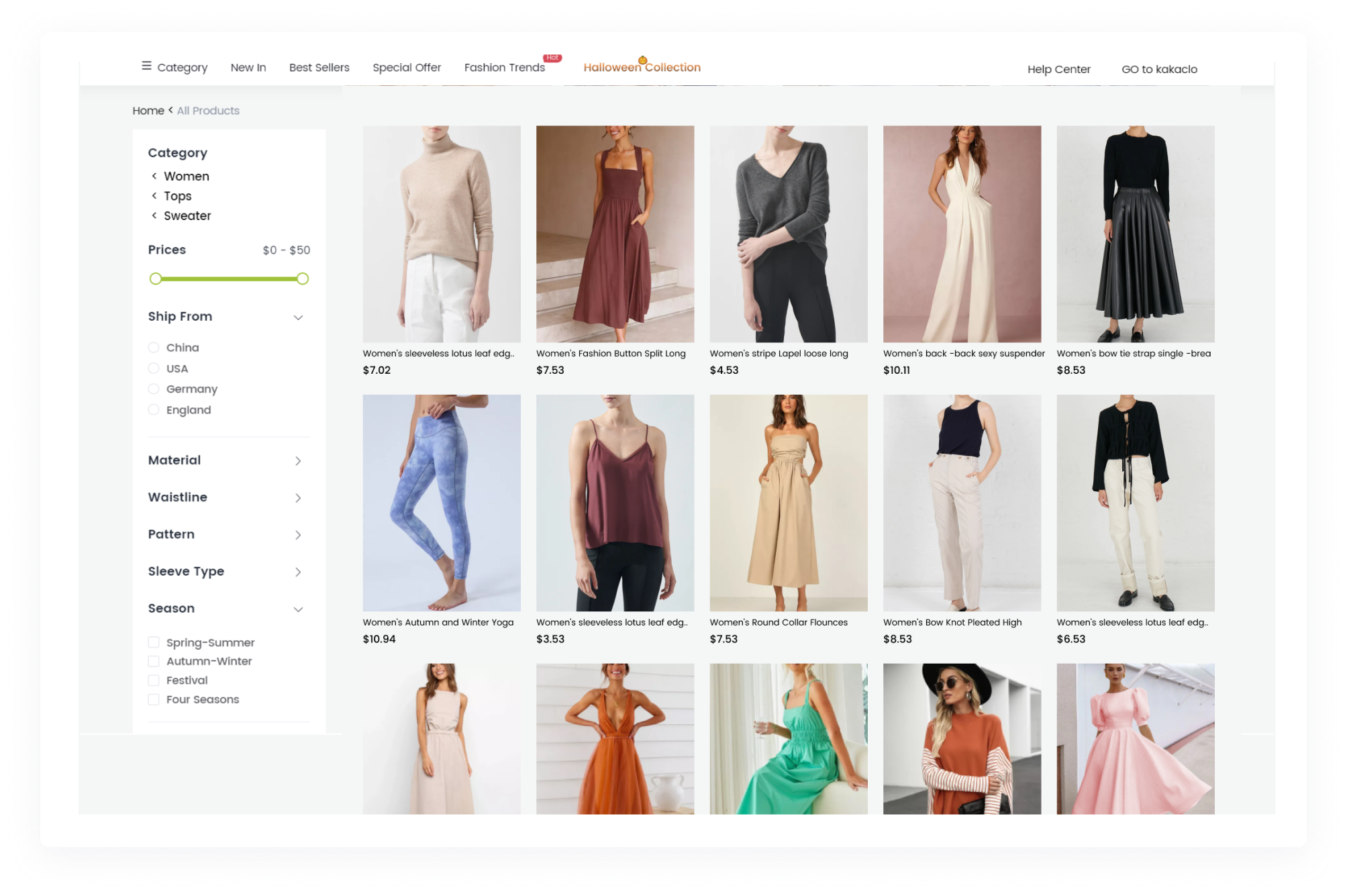The screenshot displays a detailed interface of an online clothing store. At the top of the image, there is a navigation menu with buttons labeled "Category," "New In," "Best-Sellers," "Special Offer," and "Fashion Trends." Above this menu, a prominent red button reads "New." Further down, the interface features a highlighted "Halloween Collection" in vibrant orange. On the far right, there is a "Help Center" link. 

The menu on the left side of the screenshot includes filter options titled "Category," "Women's," "Women Tops," "Sweaters" (none of which are selected), and a price range slider set from zero to fifty. Additional filters for shipping origins include China, USA, Germany, and England, along with categories for material, waistline, pattern, sleeve type, and season (with sub-options for Spring, Summer, Autumn, Winter, Festival, and Four Seasons).

The main content area showcases an array of women's clothing items. There are three rows, each displaying five different products. The selection includes various styles such as sleeveless tops with lotus leaf edges, button-split long dresses, striped lapel loose long tops, and backless designs. The apparel ranges from dresses and pants to leggings and shorts, emphasizing a broad spectrum of women's fashion.